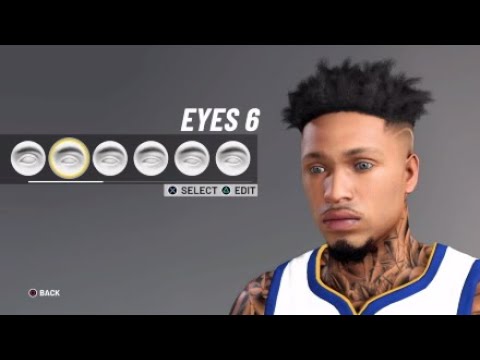In this image, we are viewing a screenshot featuring an AI-generated likeness of a handsome young man. A thick black banner runs horizontally across the top of the image, devoid of any text or graphics. Beneath this banner, the background transitions to a gray shade. Positioned centrally, the AI image portrays the young man from the chest up, clad in a white sports tank top, reminiscent of basketball attire. The tank top is accented with blue borders on both the armholes and the neckline. The neckline itself is unique, starting as a crew neck and then dipping into a small V at the center, outlined further by an inner gold border.

The young man has dark skin and sports a modest goatee complemented by a thin mustache. His hairstyle is notably stylish, with the left side of his head shaved. He appears slightly turned to the right, his profile forming a subtle, upside-down U shape. On the left side of the image, a selection menu is visible, offering a variety of options for eye shapes, presumably for editing the AI-generated face.